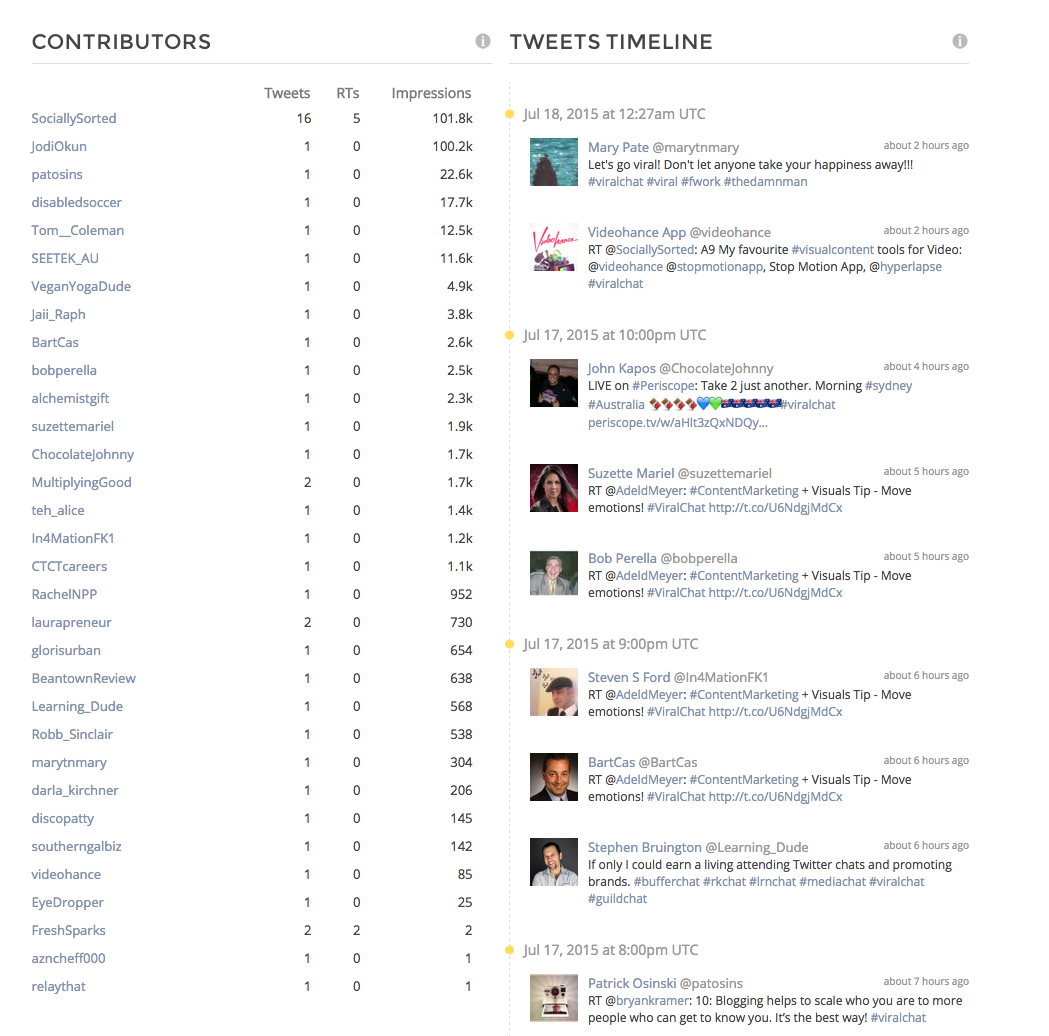The image is divided into two columns. The left-hand column is labeled "Contributors" and the right-hand column is labeled "Tweets Timeline." Under the "Contributors" section, a gray line delineates the heading from the list below. This section displays a list of 32 names, each associated with additional statistics, including tweet counts (capital "RTs") and impressions. 

The "Tweets Timeline" section includes four entries marked with yellow dots, signifying specific tweet activity dates between July 17 and July 18, 2015. The details are as follows:

- July 18, 2015: Two entries.
- July 17, 2015: Three entries visible, with one additional entry partially cut off.

At the very top of the timeline, under the date of July 18, 2015, there is a blue square marking a significant event or tweet.